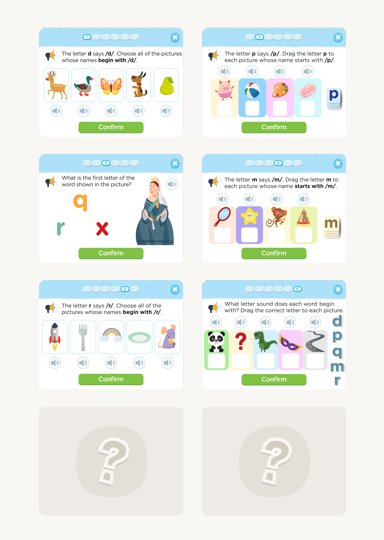Here's a refined and detailed caption based on your description:

---

"This screenshot showcases an interactive and colorful educational game aimed at children. The interface resembles a website but functions as a learning exercise platform. The main screen displays two columns of questions, each arranged in vertical sets of four squares. 

In the upper left square, the question prompts the children to identify images whose names start with the letter 'D'. The choices include pictures of a deer, duck, butterfly, dog, and pear, with the correct answers being the deer, duck, and dog. A green 'confirm' button is present for users to submit their responses and receive feedback.

Below this, another question asks, 'What is the first letter of the word shown in the picture?' accompanied by an image of a queen. Available options are 'R', 'Q', and 'X', with 'Q' being the correct choice.

Overall, the game is designed to teach children vocabulary and letter recognition through engaging and visually appealing activities."

---

This caption clearly describes the purpose and functionality of the game, highlighting its educational value and interactive elements.